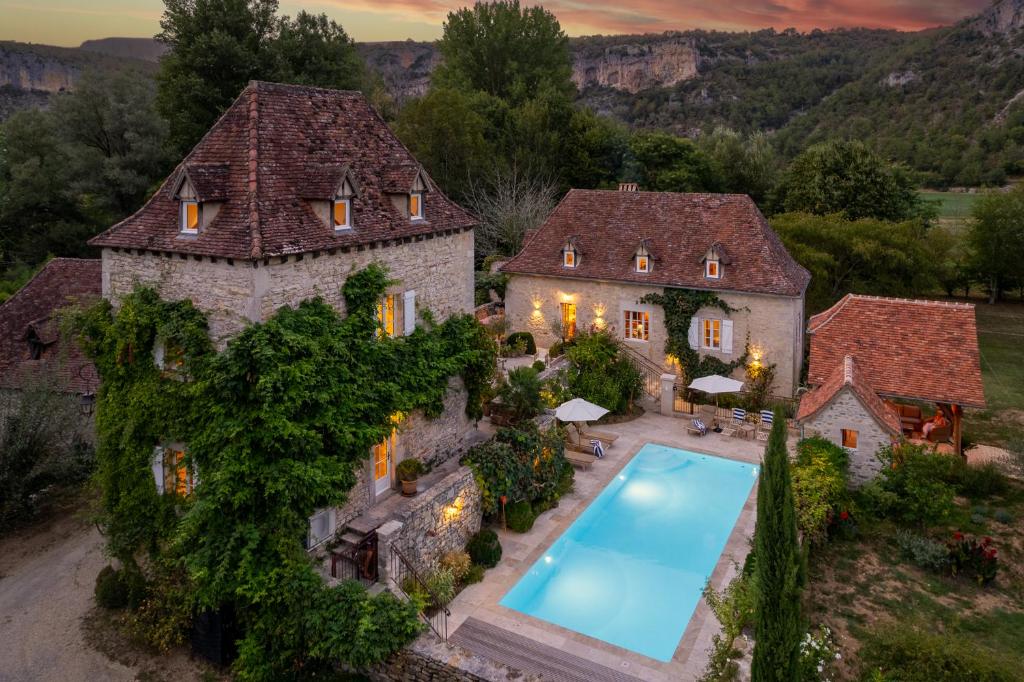A striking dusk photograph captures a sprawling mansion with an impressive architectural design, featuring sloping and gable roofs in a charming red hue, and walls in a beige or white color. To the left stands the large main building covered in lush ivy, while to the right are smaller adjoining structures, suggesting a cohesive yet diverse estate. The scene is set against the backdrop of verdant fields and gently rolling green hills, with an outcrop visible on the hillside. A vibrant, rectangular swimming pool with turquoise-blue waters lies in the foreground, surrounded by elegant potted plants, shrubs, and a notable conifer tree. The property exudes a serene yet grand atmosphere, illuminated by warm orange lights streaming through the windows and casting a glow on the vine-clad walls. A white umbrella canopy shelters outdoor furniture, adding a touch of elegance and inviting relaxation. This idyllic scene, reminiscent of a French or Tuscan villa, is further accentuated by the soft pink clouds of the setting sun, creating a picturesque and tranquil ambiance.